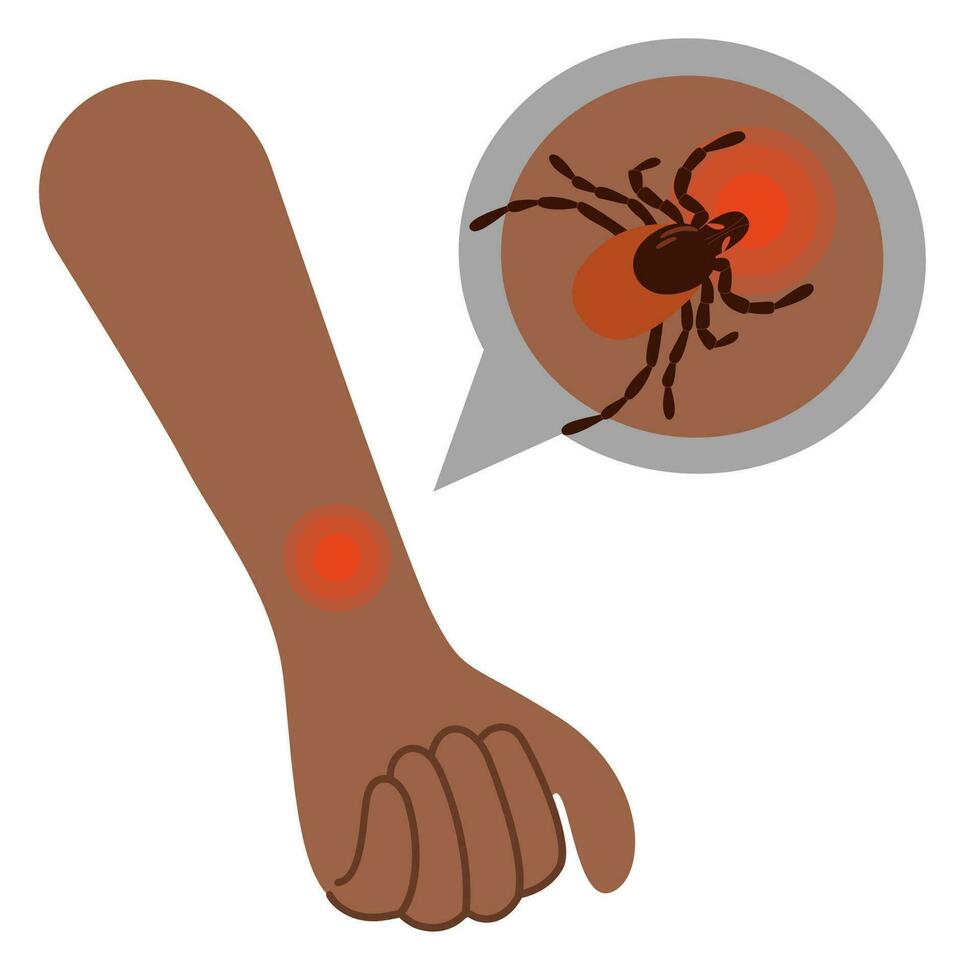This detailed infographic, designed in a cartoonish style and likely sourced from a medical pamphlet or placard, visually explains what a tick bite looks like on the arm of an African American individual. The image features an outstretched arm, depicted in varying shades of brown with detailed outlines, pointing downwards with its thumb raised. Prominently displayed on the wrist is a red bullseye mark, characterized by multiple concentric circles with progressively lighter red hues towards the outer edges.

To the right of the arm, there is a magnified view of the bullseye mark encased within a circular box, connected by an arrow pointing to the affected wrist area. This zoomed-in section, framed like a word balloon or dialogue bubble, prominently shows a graphical representation of a black and orange tick with eight legs. The tick is shown actively biting into the central, darker red part of the bullseye mark, illustrating the direct impact and bite site. The detailed highlighting of the tick-infected area in both the main and zoomed-in views underscores the informational and educational purpose of this medical infographic.